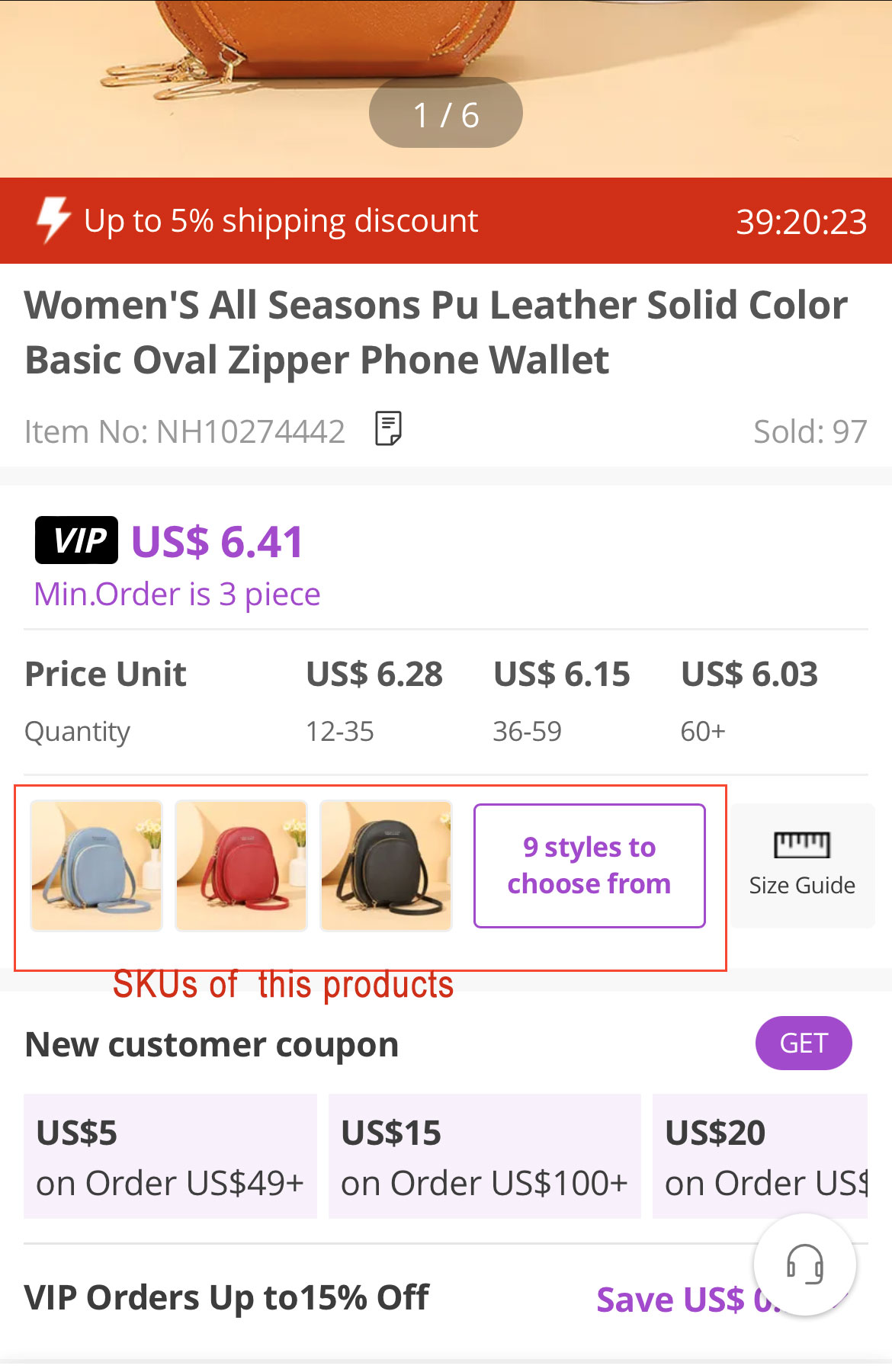This image displays a comprehensive product description for a women's all-season PU leather solid color basic oval zipper phone wallet. The wallet is eligible for up to a 5% shipping discount, which is available for the next 30 minutes and 20 seconds or within the next 39 hours and 20 minutes, depending on the specific promotion terms. 

The item number for the wallet is NH10274442. To date, 97 units have been sold. The VIP price for the wallet is set at $6.41, with a minimum order requirement of three pieces. Volume discounts are available, offering a price of $6.28 per unit for orders of 12 to 35 pieces, $6.15 per unit for orders of 36 to 59 pieces, and $6.03 per unit for orders of 60 or more pieces. 

There are nine styles available to choose from. Additionally, new customers can utilize a coupon for $5 off on orders of $49 or more, $15 off on orders of $100 or more, and $20 off on certain higher-priced orders. VIP customers are eligible for discounts of up to 15%.